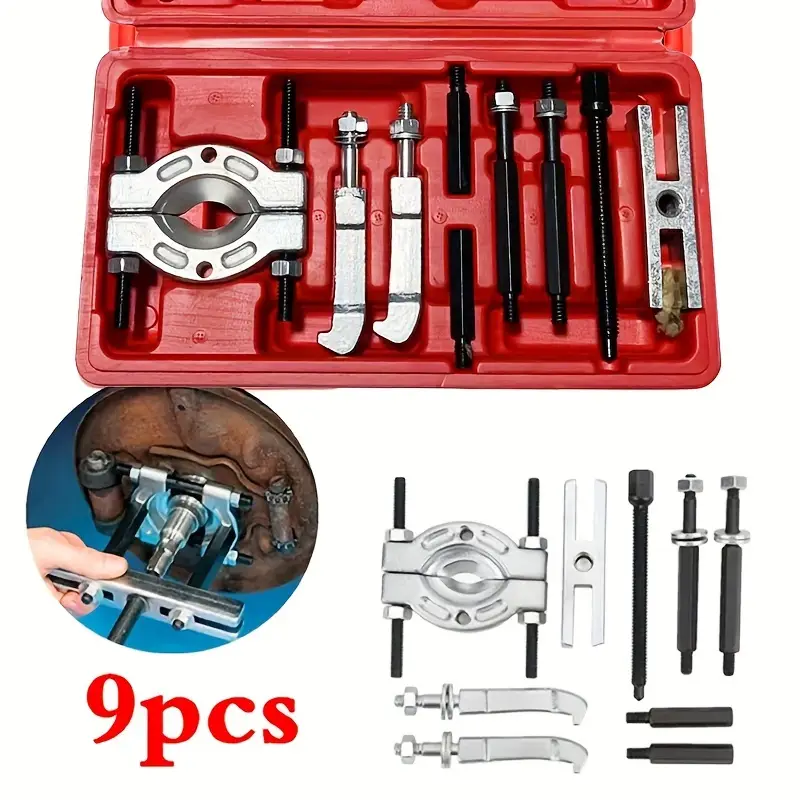The image is a detailed color photograph of a nine-piece toolkit or socket set, showcasing the product on a white backdrop, typical of commercial listings aimed at online stores, shops, or catalogs. The primary focus is a red (or orange) plastic case that holds the various components of the set, positioned near the top half of the portrait-oriented image. The lid of the case is open, though it is cropped off at the top of the photograph.

The toolkit includes several chrome and black pieces, neatly arranged inside the case and labeled "9 PCS" in red text at the bottom left. Specifically, there are two semicircular, chrome clamps with bolts and nuts positioned on the left side of the case, followed by other chrome pieces with white curved handles. On the right, there are four black pieces with nuts and bolts at each end, and adjacent to these is a silver, H-shaped object.

Below the main image of the case, the components are laid out individually against the white background to showcase each piece clearly. Additionally, the bottom middle left features a circular inset photo demonstrating the toolkit in use. This inset shows a hand actively engaging with the tool, attaching it to a vertical, circular surface, thereby illustrating the product's practical application. The photo is rendered in a style that emphasizes realism and a clear, organized layout to appeal to potential buyers.